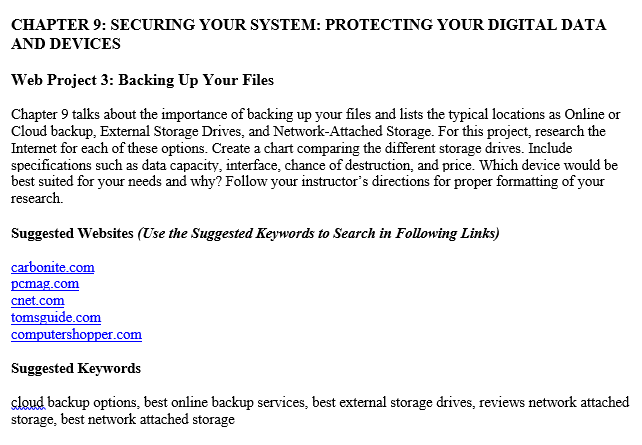**Image Caption: Chapter 9 Overview - Securing Your System and Backing Up Your Files**

This digital image features text from Chapter 9 of a web project guide focused on securing digital systems and protecting data. The chapter emphasizes the importance of backing up files and describes typical backup locations, including online or cloud storage, external storage drives, and network-attached storage (NAS).

The project assignment involves researching these backup options online and creating a comparative chart. The chart should detail key specifications such as data capacity, interface type, destruction risk, and price for each storage solution. Students are asked to determine which device best suits their needs and explain their choice.

For proper formatting and research, students should follow their instructor’s guidelines and refer to suggested websites like Carbonite.com, PCMag.com, CNet.com, Tom's Guide.com, and ComputerShopper.com. Recommended keywords for efficient search include "cloud" and "backup options."

Overall, this chapter provides essential information and resources for choosing the most suitable backup method to ensure data protection and system security.